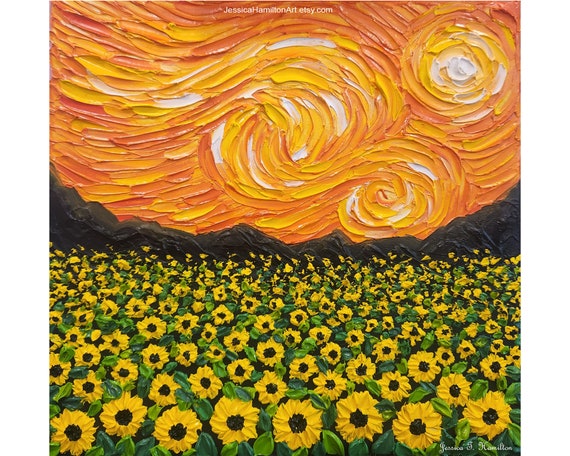The image depicts a vibrant and expressive square painting, likely an artistic rendering rather than a lifelike representation. The bottom half of the canvas is dominated by a field of sunflowers, which are painted with yellow petals and black centers, set against green leaves. Above the sunflowers rises a dark, jagged mountain range, depicted in shades of brown to black, suggesting distance and depth. The sky above the mountains features three prominent swirls of yellow, red, orange, and white, reminiscent of the dynamic patterns in Vincent van Gogh's "Starry Night," emphasizing a sense of movement and emotion. The texture of the paint appears thick, indicative of oil painting, with a smudgy, less detailed style. In the top right corner, the artwork is signed with the text "jessicahamiltonart.etsy.com," and another white text towards the right-hand side reads "Jessica [something]".